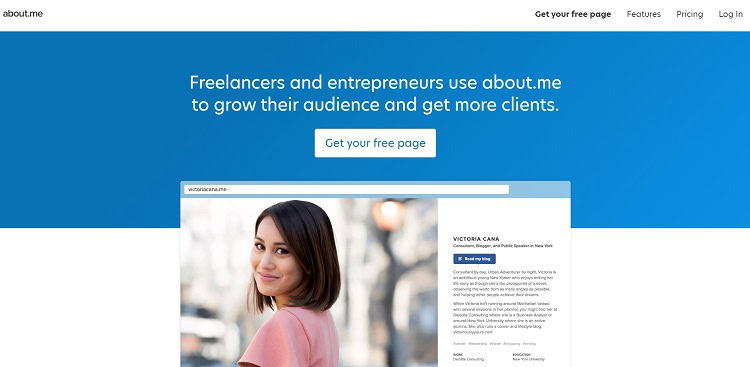The image is a polished, colorful landscape screenshot of an about.me web page. At the top right, several tabs are visible: "Get Your Free Page," "Features," "Pricing," and "Login." The current tab selected is "Get Your Free Page." Dominating the upper section is a large blue banner with white text that reads, "Freelancers and entrepreneurs use about.me to grow their audience and get more clients." Beneath this statement is a prominent white button labeled "Get Your Free Page." Additionally, the page displays an example of what a free page could look like.

The example free page showcases a professional-looking photo of a woman in her late 20s or early 30s. She has medium-length brown hair that reaches her shoulders and is wearing a pink blouse. The photo is sharp with a deliberately blurred background, enhancing its professional quality. Her face is clearly visible, giving the impression of a polished and well-crafted page. The page also includes her name and a short bio description.